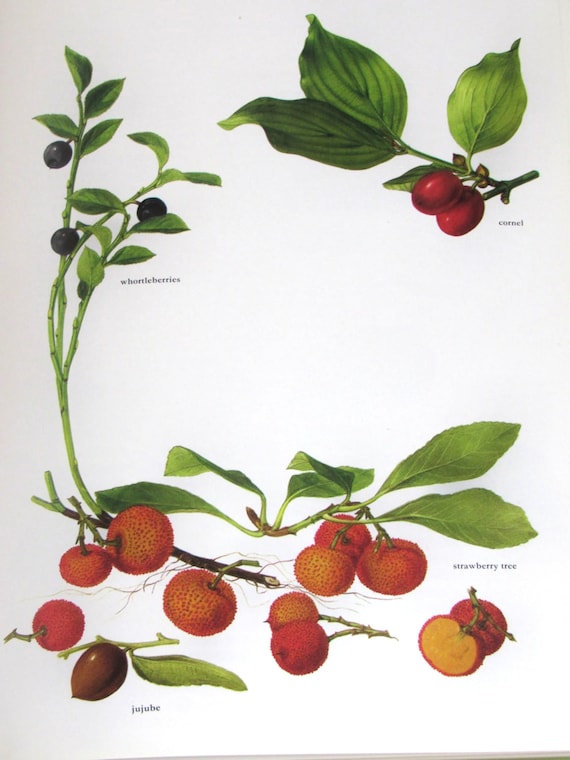This image is a detailed, artistic illustration, likely done in watercolor on watercolor paper, depicting four different types of fruits against a white background. The illustration is arranged mainly around the edges, with each fruit occupying a distinct quadrant. 

In the top left quadrant, there are wartleberries, characterized by their dark blue color, hanging off green stems with green leaves. In the top right quadrant, the image shows cornet berries, resembling the size of grapes and colored red, also hanging from green stems with multiple green leaves. Moving to the bottom left quadrant, a brown, acorn-sized jujube is depicted, attached to a green stem alongside a single leaf. The bottom right quadrant features a spiky, reddish-orange fruit identified as part of a strawberry tree; this fruit is shown cut in half, revealing a yellow interior. The illustration focuses on the intricate details of each fruit, their stems, and leaves, aiming to provide a clear and informative visual guide.